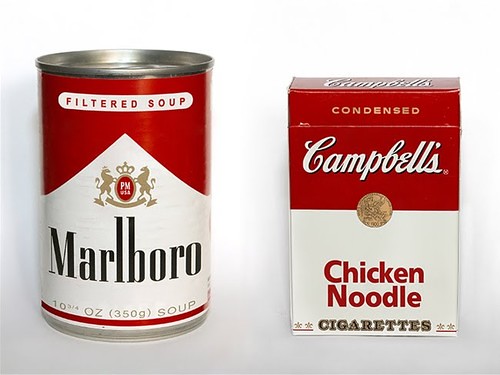In this surreal and thought-provoking image, a can of Campbell's noodle soup and a box of Marlboro cigarettes have undergone a creative logo swap. On the left, a metal can of soup is prominently displayed. It features a label with the text "Filtered Soup" at the top and the iconic Marlboro logo just below it. The can also specifies that it contains 10 3/4 ounces or 350 grams of soup. On the right, a box of cigarettes showcases the Campbell's logo both at the top and on the lid of the box. The label reads "Condensed Campbell's" with "Chicken Noodle Cigarettes" beneath it. Both the soup can and the cigarette box are adorned with classic red, white, and black designs, accented with subtle gold elements that are characteristic of their respective original brands. This clever and detailed image blurs the lines between consumer products, making a playful commentary on branding and product identity.